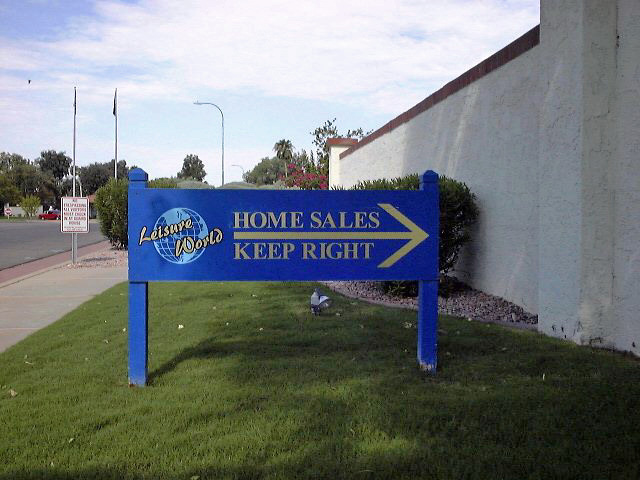The image features a large, blue sign situated on a lawn, intended to direct vehicular traffic. The sign prominently displays the message "Home Sales, Keep Right" in yellow font. Below this message, the words "Leisure World" are written in elegant cursive script, also in yellow. Behind the cursive text is an illustration of a globe. 

The background includes a concrete wall typical of the architectural style found in Nevada or Arizona. The sky is clear, indicating a bright daytime setting. Below the sign, near a curved edge with a distinct red trim, there is a white sign that appears to offer further directions. Adjacent to this area is an open parking lot, visible in the scene.